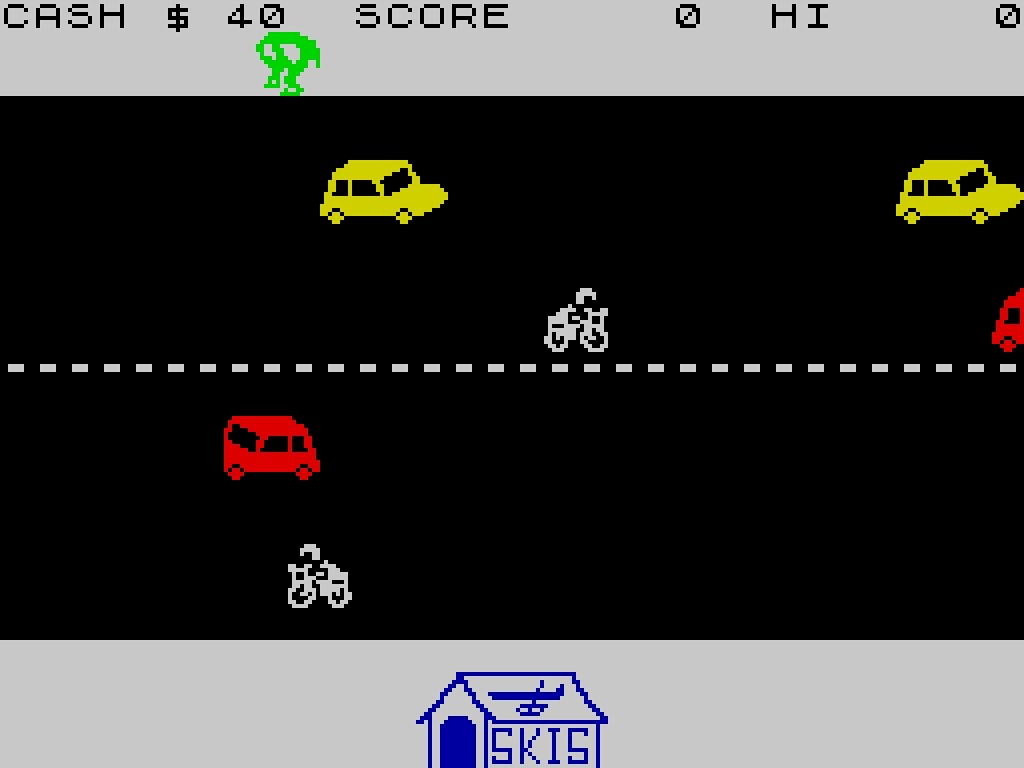The image depicts an 8-bit or 16-bit, 2D racing game reminiscent of Frogger. At the top of the screen, in black letters, it reads "Cash $40, Score 0, High 0" alongside a small green character. The gameplay area resembles a road with a horizontal white dotted line running through the middle, creating a clear division. On the upper half of the road, two yellow cars, a partial red car, and a white motorcyclist with a white helmet are visible. Similarly, on the lower half, there is another red car and a white motorcycle. The bottom and top of the screen feature gray strips. Additionally, at the bottom, there is an image of a blue house with a blue door labeled "skis" in blue letters.